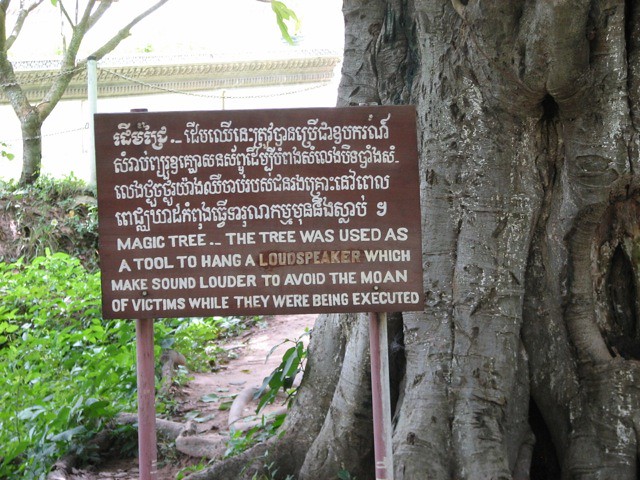The photograph, taken outdoors during the daytime, features a massive, old tree with a thick, knotty gray trunk that dominates the right half of the image, stretching from top to bottom. On the left side, partially obscured behind the tree, a wooden bridge or intricately designed wall stands out with its elaborate, yet indistinct carving due to the distance. The scene is brightly lit, suggesting a clear, sunny day. In front of the large tree, a wooden post supports a brown rectangular sign with text in both a foreign script and English. The English portion reads: "Magic Tree. This tree was used as a tool to hang a loudspeaker which makes sound louder to avoid the moan of victims while they were being executed." Below the sign is a patch of green grass, interspersed with dirt and vines. Further to the left in the background, a slender, nearly leafless tree stands beside a chain or rope fence, beyond which another structure or possible body of water can be faintly seen. The base of the large tree also shows several knots and holes, adding to its ancient and weathered appearance.